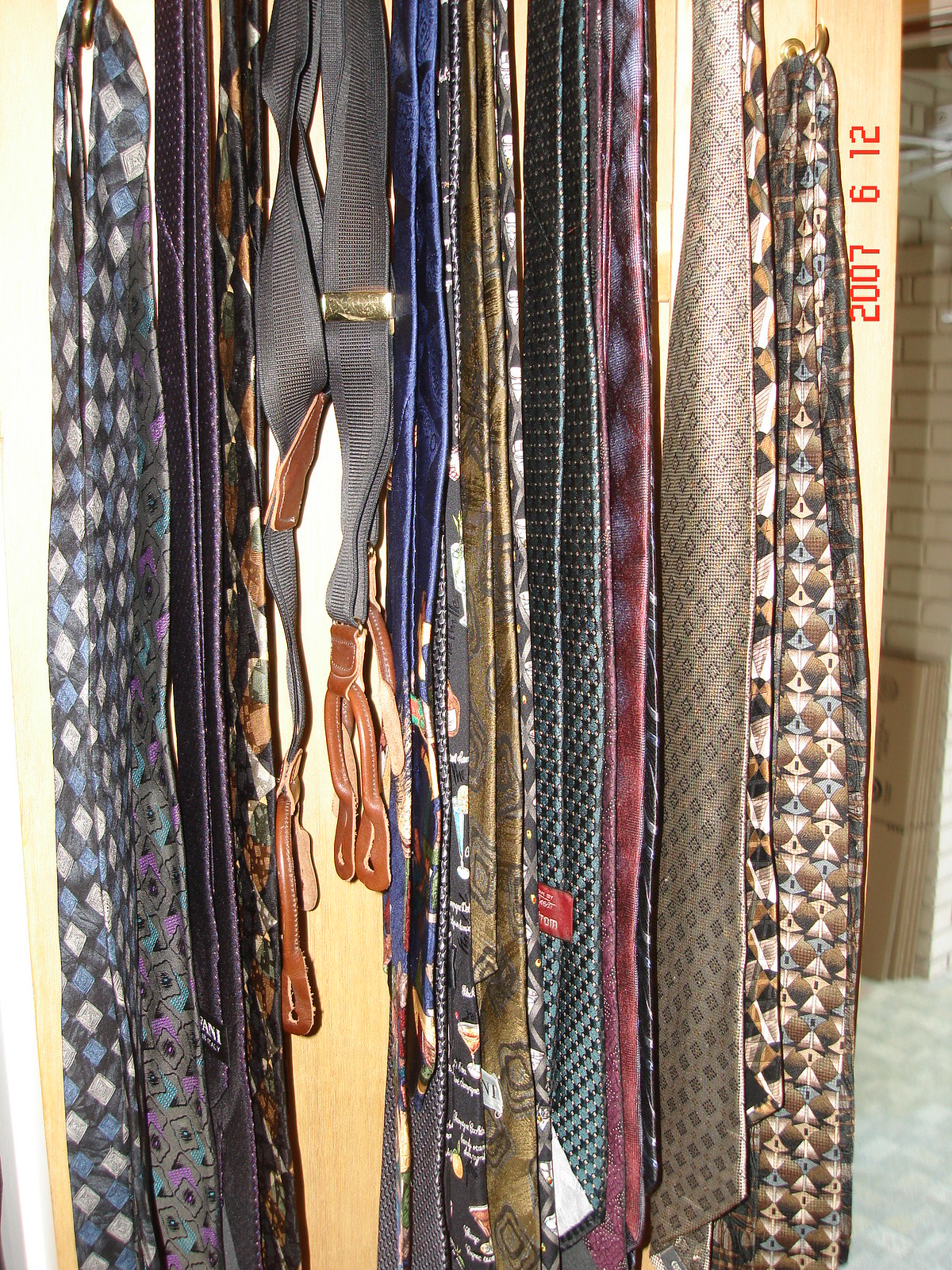The image is a photograph showcasing a collection of ties and suspenders, presumably hanging in a closet. The background is a plain gray floor, and on the far right, a light brown wall shows the date "2007-6-12" in red print, aligned vertically. The ties are hanging vertically from the top, with their tops and bottoms cut off from the frame, and appear long and varied in design.

Starting from the left, the first tie features a diamond pattern in blue and off-white. Moving right, there is a black tie followed by another black tie with a possible gold pattern. Continuing, a set of gray suspenders with brown leather attachments is visible. Next, a dark blue tie is seen, followed by a black tie adorned with images resembling beer or wine glasses. A gold tie with a black design comes next, succeeded by another gray tie displaying black diamonds. Further to the right, ties of burgundy, gold with black diamonds, and brown with gold and off-white hourglass shapes are discernible. 

Additional descriptions highlight ties with abstract patterns and darker colors, including purple, aqua, blue checkered, red checkered, and a reddish tie that appears patternless. Overall, around 11 or 12 ties can be counted. Despite varying color descriptions—a mix of browns, dark blue, dark gray, and muted tones—the consensus indicates the ties originate from either a man's personal collection or possibly a store display. The presence of suspenders and the closeness of the ties suggest a personal, perhaps meticulously organized, collection.